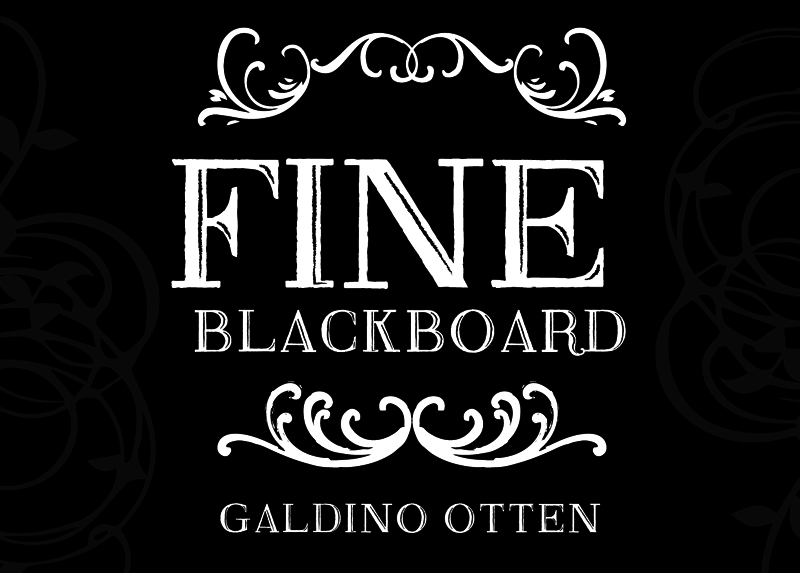The image is a striking black and white advertisement that appears to be promoting something related to a restaurant or theater. The background of the sign is a deep, solid black, creating a bold contrast with the white text. The sign's layout is vertically centered with intricate decorative designs at the top and bottom. These designs are composed of elegant, swirling, or curly-cued patterns reminiscent of connecting swan heads forming swooshes, which give the advertisement a classy and refined look.

At roughly the upper third of the image, the word "FINE" is prominently displayed in large, capital letters. Below this, in smaller yet still noticeable white font, is the word "blackboard." These words are perfectly centered within the image, positioned between the ornate decorative elements.

Further down, at the bottom of the sign, the name "Galdino Otten" is clearly spelled out in white, adding to the overall visual balance of the design. This sophisticated and visually appealing layout strongly suggests a high-end advertisement, possibly for a fine blackboard product or a related service by Galdino Otten.